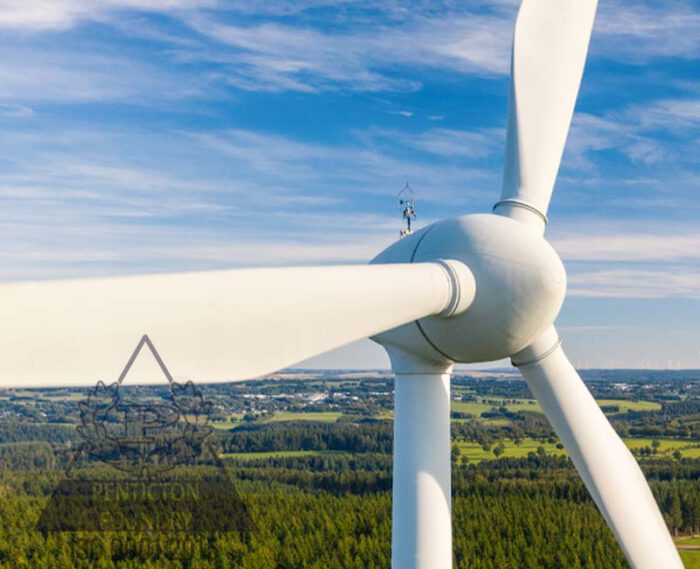The image showcases a close-up view of a white windmill with three long blades centered around a round dome-like hub. The windmill is mounted on a white pole and is slightly turned to the side. Atop the windmill, there's a tiny figure, possibly a construction or maintenance worker. The background features a beautiful, mostly clear blue sky with a few white wispy clouds and extends to a horizon filled with densely packed green pine trees and patches of grass. To the bottom left of the image, there is a semi-transparent logo with a triangle outline and a large "P," accompanied by the text "Penticton Foundry.” Also visible in the distance are traces of a village with buildings scattered among the natural landscape.